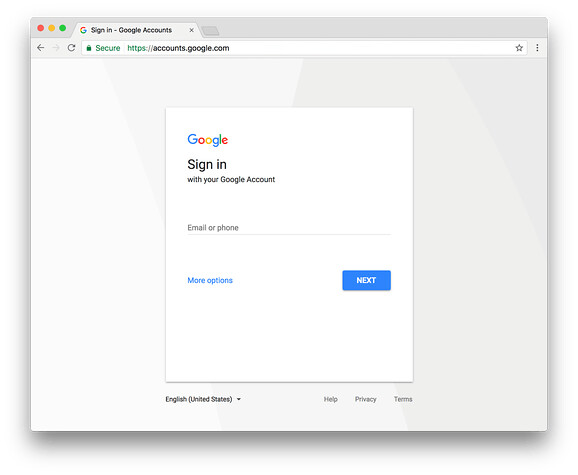The image is a screenshot of a computer screen, likely from a macOS device evidenced by the distinctive red, yellow, and green circles in the top left of the window. The open window displays a tab filling the entire screen. The tab is for a Google sign-in page, as indicated by the Google logo and the text "Sign in - Google Accounts" at the top. Below, the URL bar features the secure HTTPS address "https://accounts.google.com" and an unfavorited star icon on the right side. The main content of the page is a large white square inviting users to "Sign in with your Google Account." Beneath this prompt, there are fields to enter an email or phone number, accompanied by a "Next" button for proceeding to the password entry step. The overall color scheme of the page is predominantly white and light gray, and there are no other tabs open. At the bottom of the page, there are links for "English (United States)," "Help," "Privacy," and "Terms."